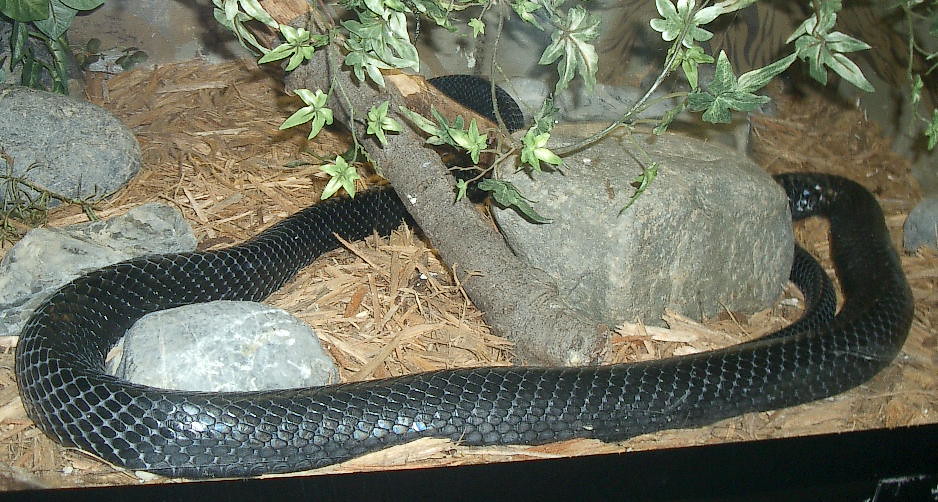The image depicts a large, black snake with glossy scales, partially coiled around a central rock inside a glass terrarium. The snake’s body, which appears grayish black, is wrapped in a horizontal manner, intertwining around a considerable rock situated in the center and another gray rock with white stripes at the lower left corner. The snake's surroundings include a variety of landscape details: towards the right of the snake, there is another rock, and a branch extends to the left, accompanied by green leaves and some green twigs adorned with white petals. The terrarium's ground is covered with a mix of brown wood chips, bits of straw, and dirt. The black edge of the terrarium is visible at the bottom, framing the earthy setting that houses a total of three notable rocks. The scene vividly portrays the snake in its enclosure, creating an almost intimidating sight.